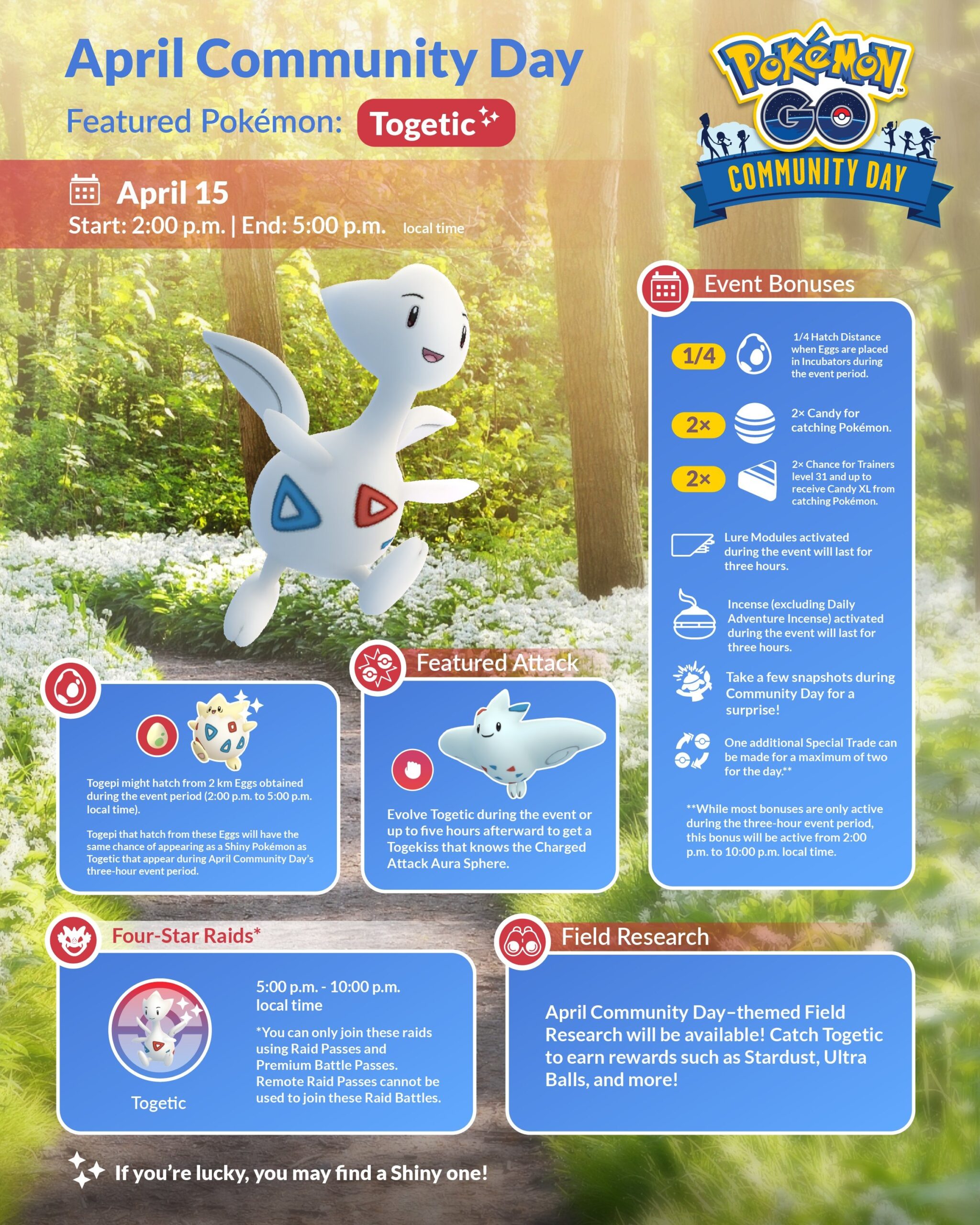The image is a promotional webpage for Pokémon GO's April Community Day event, featuring a lush forest background with vibrant green trees, brown trunks, and a scattering of white floral plants. Dominating the visual is an evolved form of Togepi, known as Togetic, presented either as an evolution or possibly a fusion with another Pokémon.

At the top of the page, under the shining sun overlaying a translucent rectangle, the event title "April Community Day" is boldly displayed in dark blue. Beneath it, in matching dark blue text, is the phrase "Featured Pokémon." Below this heading is an oval button with white text reading "Togetic," flanked by three stars.

On the right side of the webpage, the iconic Pokémon GO logo is prominently featured. The word "Pokémon" is rendered in yellow, outlined in blue, with an accented 'E,' while the "GO" part is a mix of dark blue and cyan, with the center of the 'O' housing a traditional Pokéball, split into red and white halves with a central white circle.

Silhouettes of people frame the scene on both the left and right sides. Across the bottom, a dark blue ribbon-shaped rectangle bears the bold yellow text "COMMUNITY DAY."

On the left-hand side, a muted, faded red rectangle contains the event details. In white text, it reads "April 15th." Below this, the schedule is outlined with "Start: 2 p.m." on one line, a separator, and then "End: 5 p.m.," indicating local time.

In the foreground, the featured Pokémon, Togetic, is showcased. This creature resembles Togepi at the base, but with an elongated face and head, white wings, arms, and legs contrasting Togepi's typical cream color. Decoratively, it has blue and red triangles on its body.